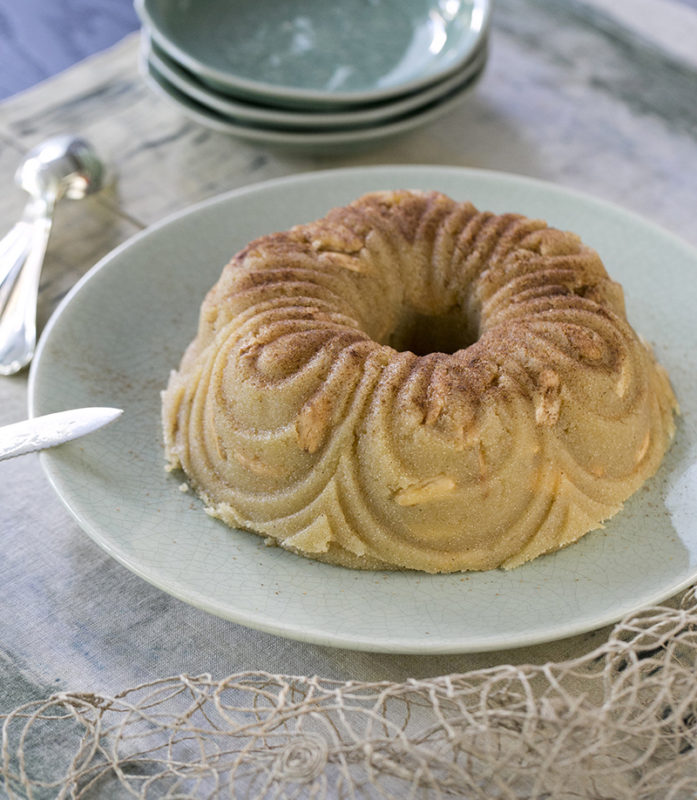A light yellow pastry, resembling a flattened donut or mini Bundt cake, sits on a light green saucer speckled with brown. The pastry features circular patterns on top and is sprinkled with brown cinnamon-like powder. An almond-like texture is noticeable on its exterior. To the left, a silver knife with a sharp point reflects white light and leans against the saucer. Above, a silver spoon also reflecting white light rests on a light gray tablecloth streaked with blue. At the top, there’s a stack of three similar saucers with teal centers and white edges. Across the bottom, a bundle of brown strings forms a web-like arrangement from left to right.